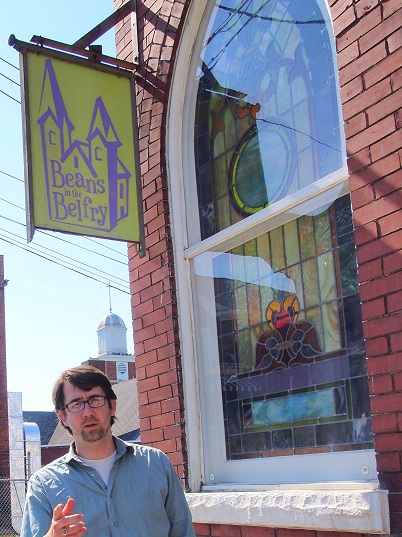In this vibrant daytime image, a middle-aged Caucasian man stands outside a red-brick building, likely a store or café. He sports a light blue button-up shirt over a white undershirt, black glasses, and a stubbled goatee. His short brown hair and pointed gesture with his right index finger add to his casual demeanor. 

Next to him is an impressive stained glass window, housed in a white frame, showcasing an array of colors—green, red, blue, yellow, and turquoise—with a distinctive circular blue piece at the top. The arched window further features a regular glass pane in front of it.

Above the man, a sign with a green flag, embellished with a purple castle logo, reads "Beans and the Belfry" on an unattractive mustard yellow background. This sign hangs from the brick building, reminiscent of a church setting. In the distant background, a white-domed chapel with a cross is visible, illuminated by the bright midday sun. The overall scene captures a mixture of the quaint and the divine, bathed in natural light.